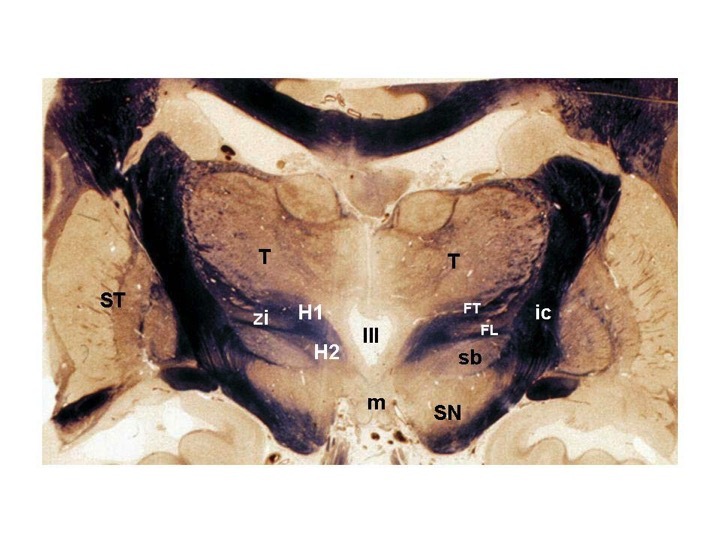This image appears to be a detailed diagram or X-ray of a pelvic skeletal structure, possibly intended for educational purposes. The background features a light tan, almost sandy color with darker brown and black accents. In the center, a darker brown hue indicates a lower, canyon-like section. The image is annotated with a combination of capital and lowercase letters throughout: notable annotations include `ST`, `T`, `zi`, `h1`, `h2`, `m`, `Sn`, `sb`, `ft`, `fl`, `ic`, and a Roman numeral `III` in the very center. The placement and combination of these letters suggest that they correspond to different areas of the skeletal structure being depicted.